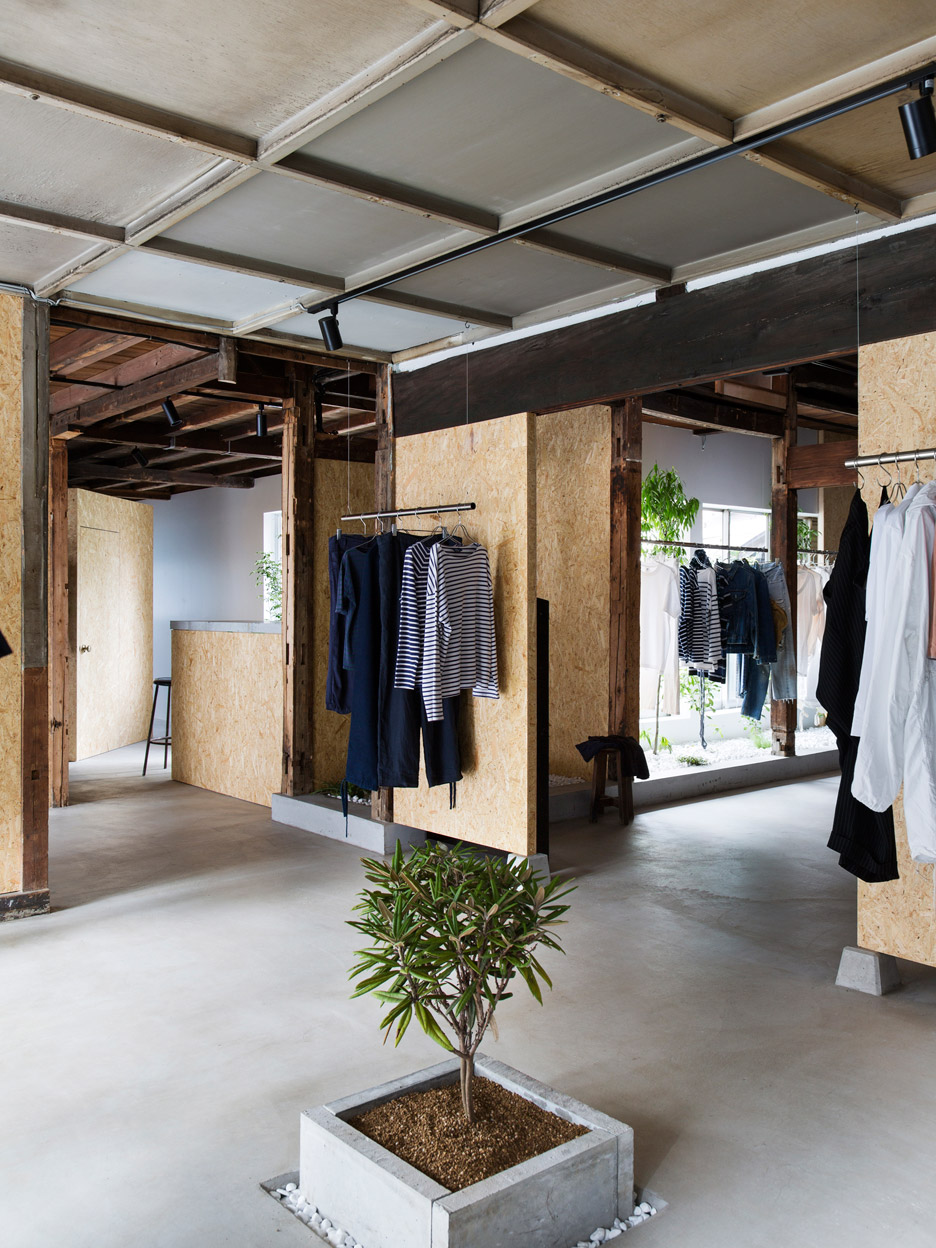The photograph captures the interior of a sparse, minimalist clothing boutique with a distinctly industrial aesthetic. The flooring is unfinished, polished concrete, and the walls are primarily bare plywood, providing a raw, utilitarian backdrop. In the center of the store, a small boxed plant sits in a square planter surrounded by white rocks, adding a touch of greenery to the space. The ceiling features a metal grid system with recessed can lighting.

Hanging from suspended metal racks are a few carefully selected items of clothing, including striped shirts, black dresses, white shirts, and jeans, hinting at a high-end selection due to the boutique's open-plan layout and minimalist design. A stool is visible off to the side, along with some hanging plants, though the store appears devoid of people. The boutique's stark, unfinished look, combined with the limited but neatly arranged clothing, suggests an expensive, curated shopping experience.